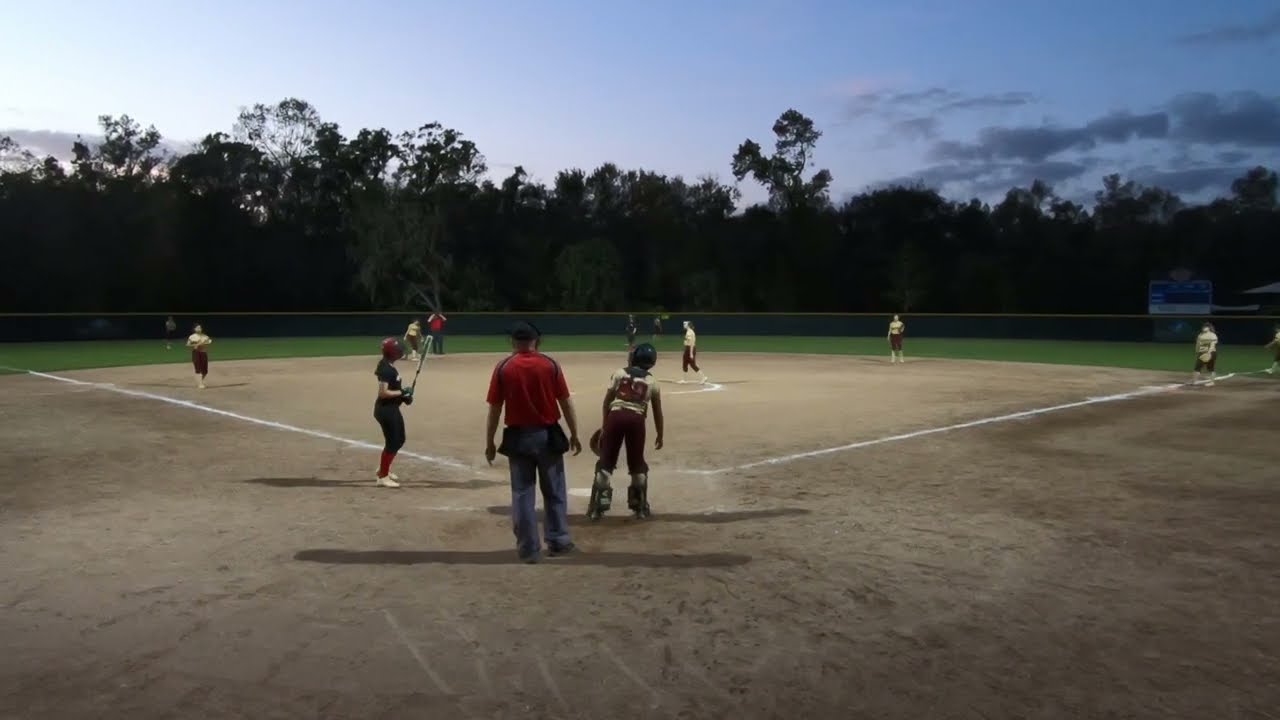In this detailed photograph, a group of young girls is playing softball on a field surrounded by lush green trees. The dirt infield and grassy outfield are bordered by a dark green fence topped with a yellow stripe. Visible on the right side are blue advertisements or possibly a scoreboard. 

The scene includes two teams, each distinct in their uniforms: one team in dark burgundy pants and yellowish shirts, and another in dark attire with red socks and red helmets. All players are equipped with helmets for safety. Among them, a girl stands confidently holding a baseball bat, ready to take her position in the batter's box.

Accompanying the players are two coaches, identifiable by their red shirts, grey or blue hats, and jeans. An umpire, donning a black hat, mask, red shirt, and grey pants, stands at the ready, overseeing the game. The catcher is in position, while the batter is preparing to step into the box.

The photograph captures the ambiance of an evening setting, with a sky painted in hues of purple, blue, and white. Clouds gather mostly on the right side, adding to the drama of the dimly lit field. The atmosphere is filled with anticipation as everyone awaits the batter's swing.